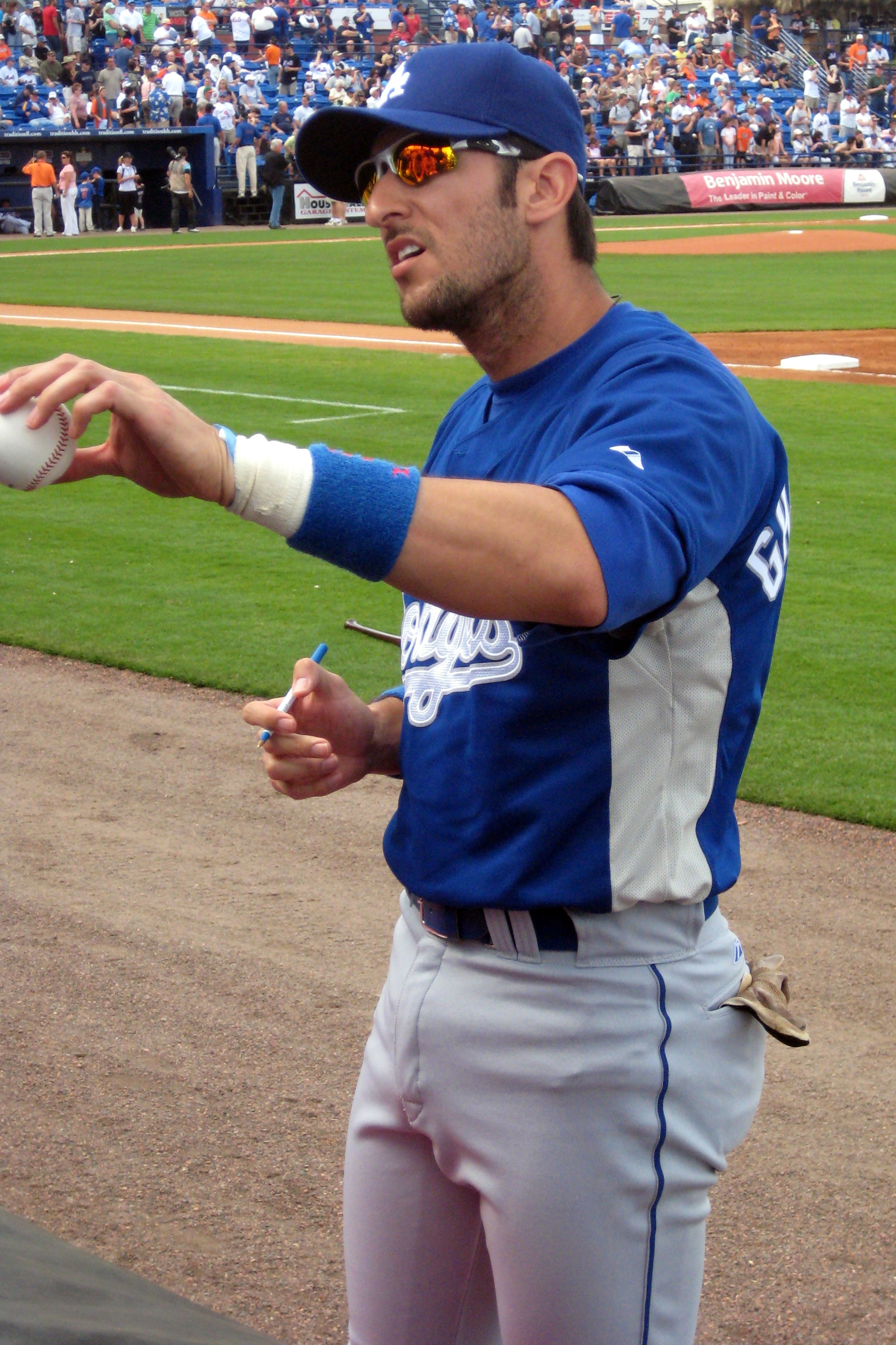The photograph captures a baseball player in the midst of signing a baseball for a fan. He is dressed in a blue and white jersey with a blue cap that features a white 'A.' The player sports gray pants and a blue belt, complemented by a blue and white wristband on his left hand. He appears to be in conversation with the fan, given his slightly open mouth displaying the top row of his teeth and his head tilted a bit to the right. A stubbly beard and mustache cover his face, partially obscured by his sunglasses. In his right hand, he holds a blue pen, while his left hand extends the baseball towards the unseen fan off-frame to the left. Behind the player, the image showcases a packed stadium with excited fans, a green and brown baseball field, and a visible Benjamin Moore sign in the upper right background.